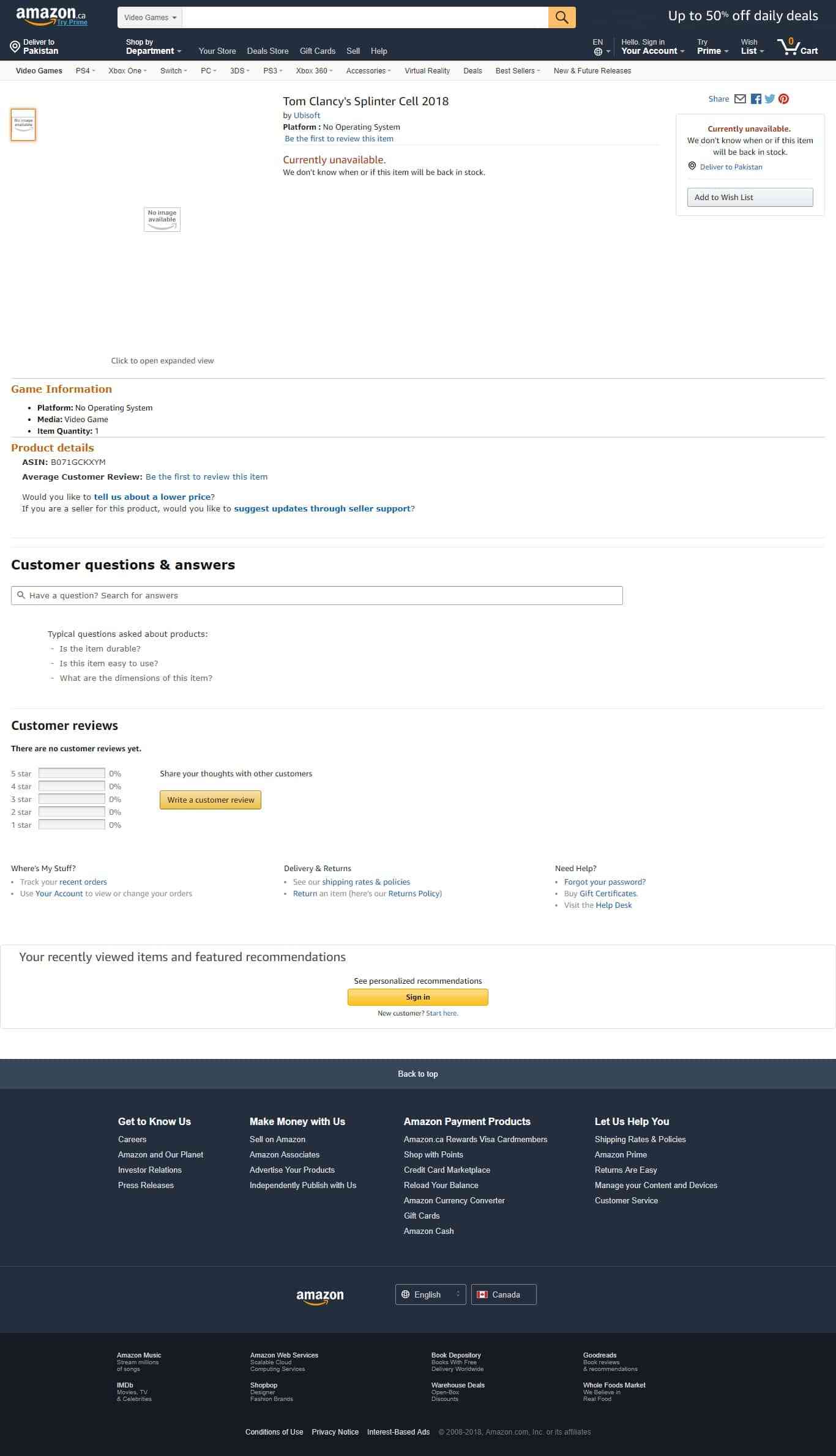The image is a detailed screenshot of an Amazon webpage displaying the listing for Tom Clancy's Splinter Cell released in 2018. At the top left corner, the familiar Amazon logo is distinctly visible, signifying the webpage's authenticity. The top navigation bar presents the standard Amazon layout: the logo on the left, followed by a centrally located search bar and an "Up to 50% Off Daily Deals" banner.

On the far left of this bar, users can see their set location, while the middle section is populated with personalized suggestions and sections based on browsing habits. To the right-hand side, quick access options for language settings, account details, Prime membership, and the shopping cart are available.

Below this navigational strip, the main content of the shopping page begins, specifically showcasing the Tom Clancy's Splinter Cell game. Interestingly, the game listing lacks an image, consisting solely of text descriptions and details that are not legible in the screenshot. 

The next section of the page features "Customer Questions and Answers," complete with an input bar inviting users to type their queries for community feedback. Following this is a segment dedicated to customer reviews, equipped with a star rating system on the left and a yellow "Write a Review" button on the right, encouraging users to share their experiences.

Near the bottom of the page, a prominent yellow sign-in button is visible, urging users to log in for a more personalized experience. Finally, the very bottom of the page contains the usual boilerplate content such as terms and conditions and agreements, often overlooked by users. 

All these elements are set against a backdrop of a large navy blue rectangle, creating a cohesive and user-friendly interface. This screenshot encapsulates the essence of an Amazon product listing page for Tom Clancy's Splinter Cell, highlighting key navigational and interactive features.